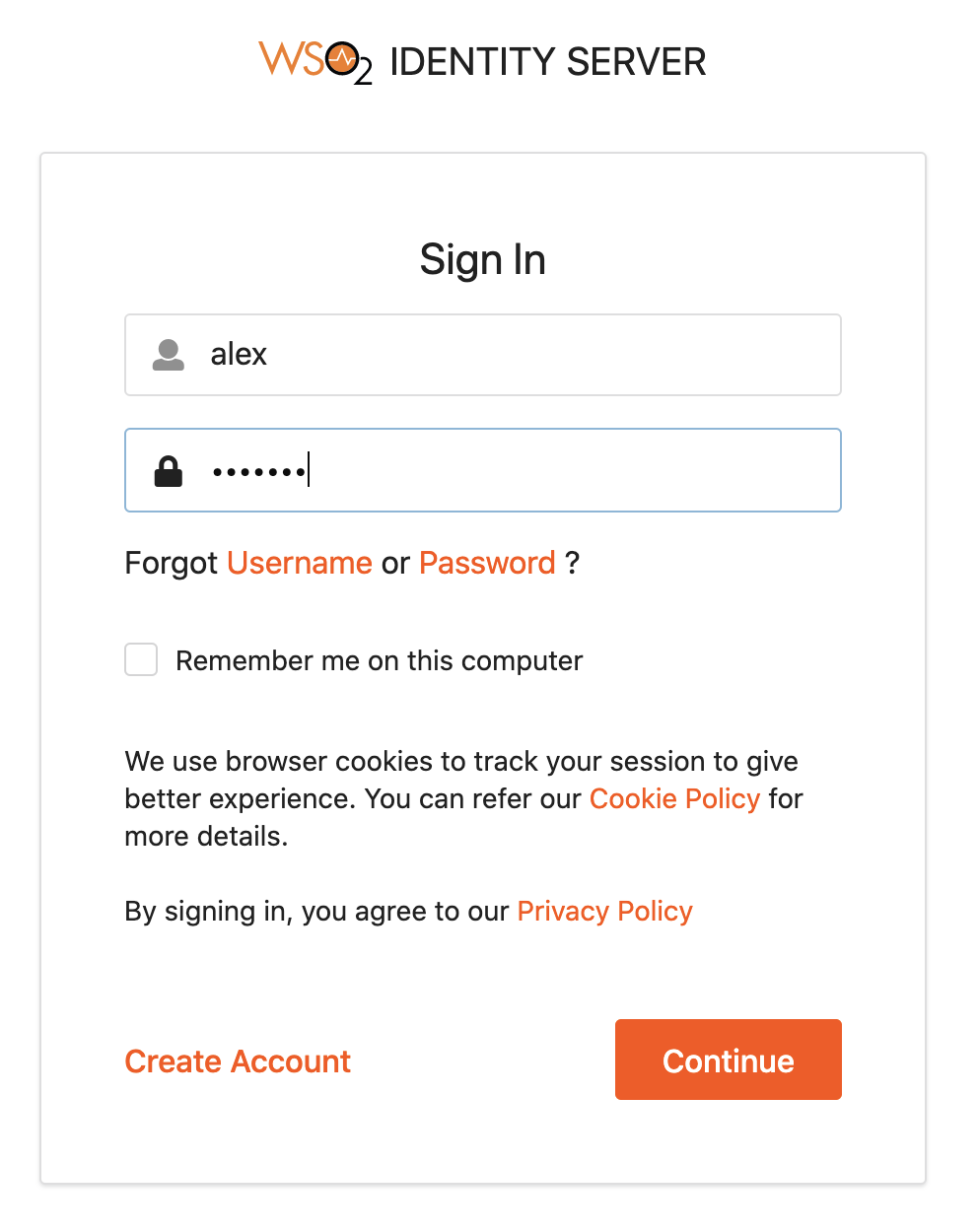Screenshot of WSO2 Identity Server Sign-In Page with Detailed Annotations

The image is of a WSO2 Identity Server sign-in page, framed by a thin gray border. The background is predominantly white, creating a clean and minimalistic look. At the top of the sign-in box, the WSO2 Identity Server logo is prominently displayed, with "WSO2" stylized in orange and black, where the "02" appears similar to the chemical symbol for oxygen, "O2".

Immediately below the logo, centered at the top, is the text "Sign In". The main content of the sign-in box starts with a gray profile icon depicting an empty figure and the name "Alex." Underneath this, there is a blue-highlighted input field containing a lock icon and concealed password dots, with a vertical cursor placed right after the last dot, indicating an active text field.

Below the password field is an option labeled "Forgot Username or Password," with "Username" and "Password" in orange and clickable. Adjacent to this, there is a selectable "Remember me on this computer" checkbox.

Further down, there is explanatory text: "We use browser cookies to track your session to give a better experience. You can refer to our Cookie Policy for more details. By signing in, you agree to our Privacy Policy." Both "Cookie Policy" and "Privacy Policy" are in orange and act as clickable links.

At the bottom left corner of the sign-in box, in larger bold font, is the text "Create Account" in orange. Finally, in the lower right-hand corner, there is an orange "Continue" button.

The remainder of the image outside this sign-in box is essentially empty white space, further emphasizing the central content.